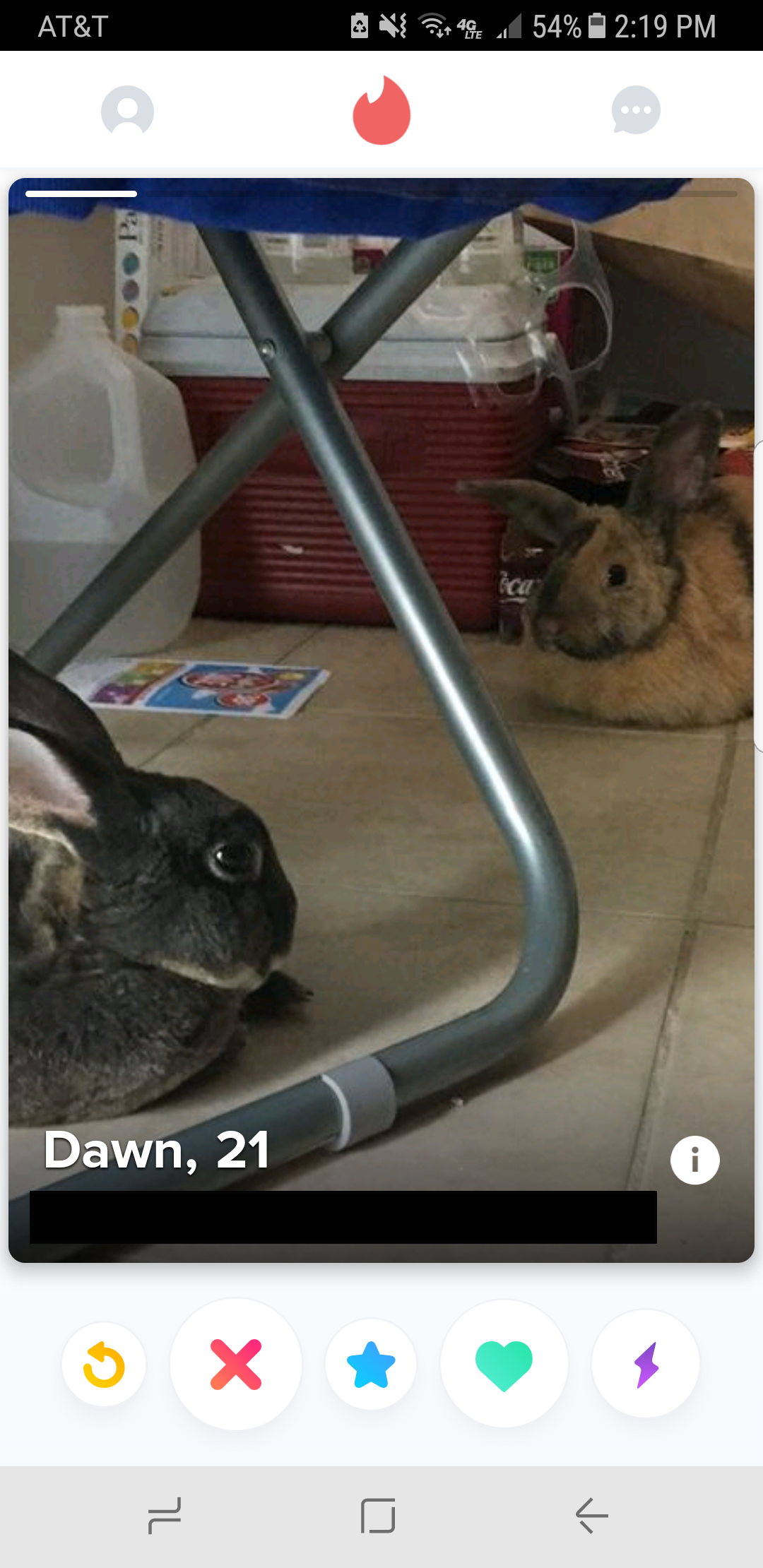A detailed screen capture of an image taken on a cell phone showcases two bunny rabbits in what appears to be a washroom with white ceramic tile flooring. The phone’s interface displays in the upper left corner that it is connected to the AT&T network with 54% battery life, and the time reads 2 p.m. In the center of the image, a dark-furred rabbit with ears pointed up faces left, exposing its right side profile. Another rabbit, situated in the upper right, has brown fur and is visible in a three-quarter view. Its left ear is pointed up while the right ear extends horizontally. 

In the background to the left of the brown rabbit is a red cooler with a white top, positioned next to a partially filled white or clear jug of water. A metallic chair leg slants diagonally from the upper part of the image into the foreground where the rabbits are seated on the tiled floor. The overlay text at the bottom left corner reads "Dawn, 21" in white font. Below this text are several icons including replay, an X, a blue star, a green heart, and a purple lightning bolt.